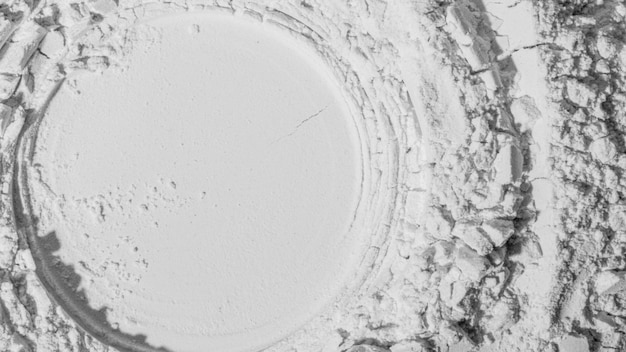The image portrays a monochromatic, close-up view of a textured powdery substance that fills the entire frame, with a white or light gray hue that could suggest either flour or snow. A distinct circular indentation appears slightly to the left, as though a round object had been pressed down into the powder. The imprint contrasts against the surrounding powder by being lightly packed, maintaining a lighter color. To the right, a vertical strip looks smoother and more compacted, creating a grayscale variation possibly due to lighting effects. Scattered throughout the surface, especially around the circle and the right side, are small specks and flecks of the powder, adding subtle texture to the image's uniform appearance. The overall impression is one of a finely detailed close-up with variations in light and texture emphasizing the powder's fine granularity.